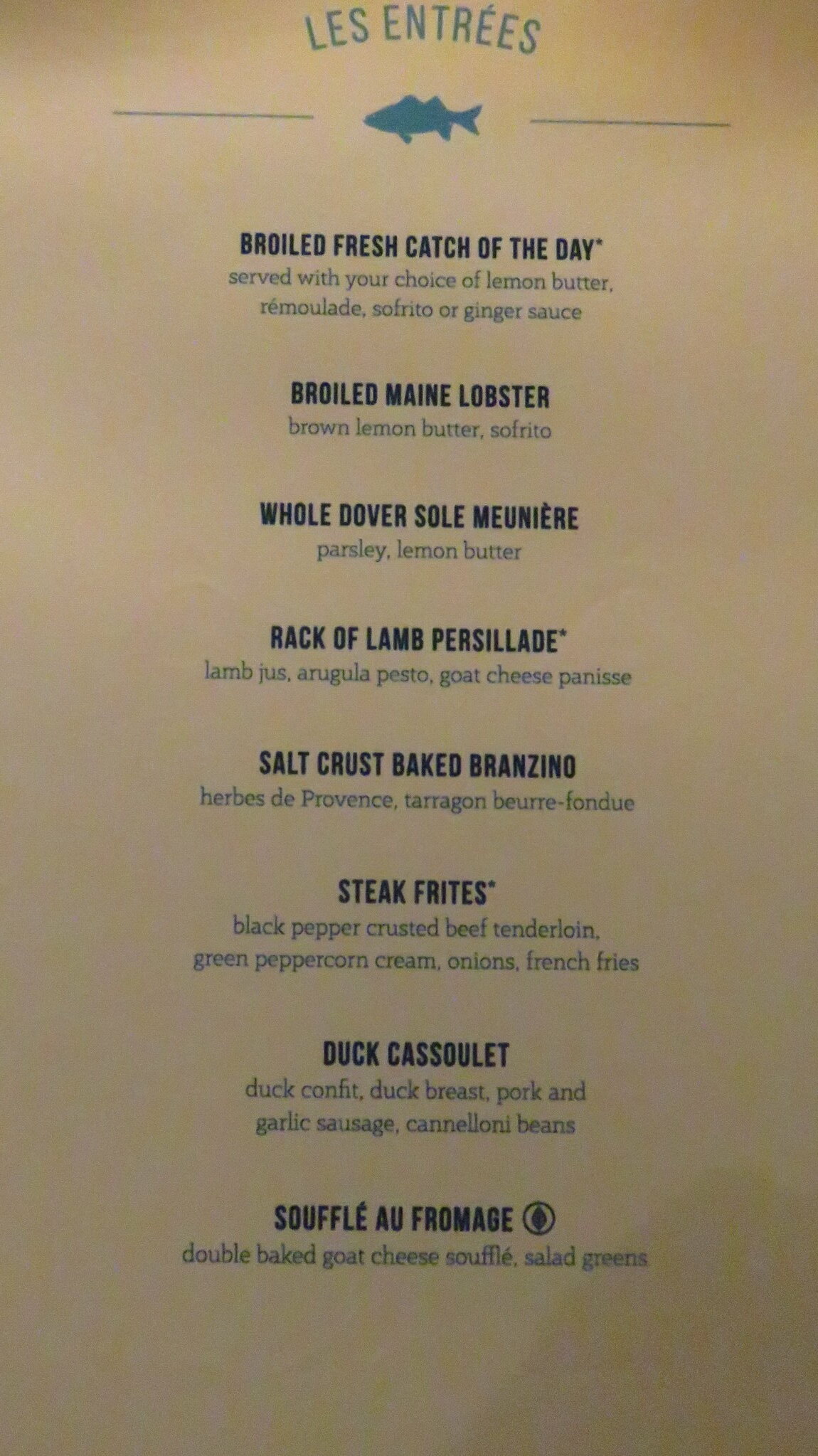This image captures a tan-colored menu page from a seafood restaurant. At the top, in elegant blue letters, it reads "Les Entrées," accompanied by a blue silhouette illustration of a fish. Below this heading, the entrees are listed in a bold dark blue font, with detailed descriptions in a lighter blue font.

The menu items include:
- **Broiled Fresh Catch of the Day**: Served with your choice of lemon butter, remoulade, sofrito, or ginger sauce.
- **Boiled Maine Lobster**: Accompanied by brown lemon butter and sofrito.
- **Whole Dover Sole Meunière**: Garnished with parsley and lemon butter.
- **Rack of Lamb**: Marked with an asterisk, this dish includes parsley, lamb jus, arugula, pesto, and goat cheese panisse.
- **Salt Crust Baked Branzino**: Flavored with herbs de Provence, tarragon, and beurre fondue.
- **Steak Frites**: Noted with an asterisk, featuring black pepper-crusted beef tenderloin, green pepper cream, onions, and French fries.
- **Duck Cassoulet**: A combination of duck confit, duck breast, pork and garlic sausage, and cannellini beans.
- **Soufflé au Fromage**: Indicated with a leaf symbol for a vegetarian option, this double-baked goat cheese soufflé is served with salad greens.

The menu is printed on a long strip of paper, offering a sophisticated and detailed selection of entrees in a visually appealing layout.